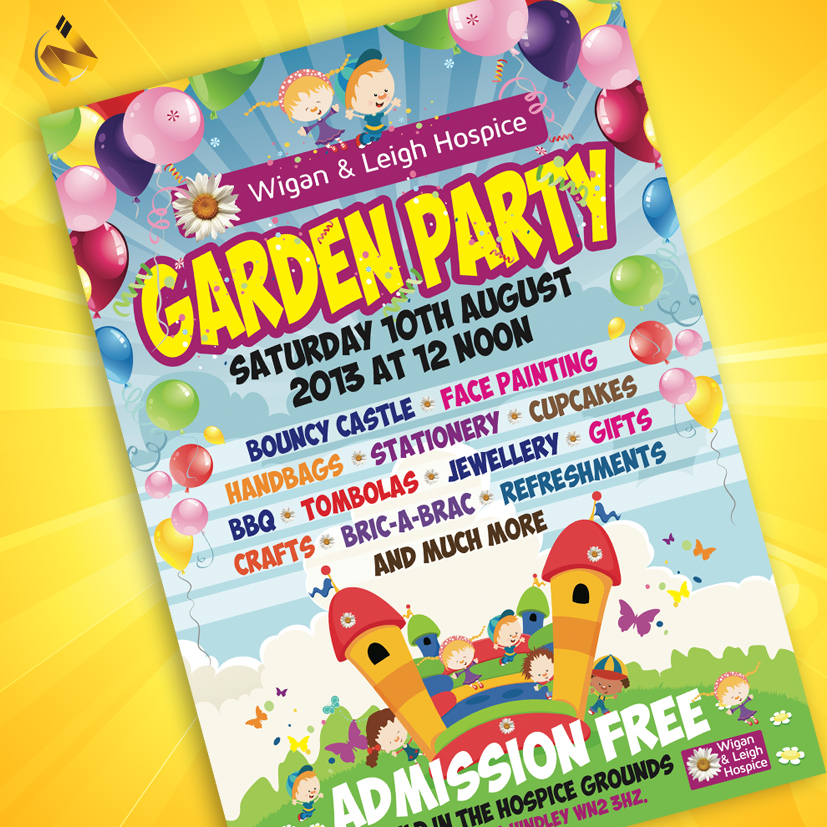The flyer, designed digitally with a vibrant yellow background featuring radiating sun rays, is displayed at an angle, with the top slanting towards the 10 or 11 o'clock position and the bottom towards the 5 o'clock position. The main elements on the tilted flyer include multi-colored balloons (pink, purple, red, blue, green, yellow) cascading from the top corners to the center, creating a festive border. At the center, a cheerful cartoon illustration depicts a young girl and boy with reddish hair jumping and playing, exuding a sense of joy. Below that, the text on a purple background reads "Wigan and Lee Hospice" with a white flower logo to the left.

In large, bright yellow text with a purple border, the flyer announces the "Garden Party" scheduled for Saturday, 10th August 2013 at 12 noon. The detailed list of activities includes a bouncy castle, face painting, handbags, stationery, cupcakes, barbecue, tombolas, jewelry, gifts, crafts, and refreshments, all mentioned in vibrant colors like blue, pink, purple, and yellow. At the bottom, another cartoon of kids enjoying a bouncy house, which features two side towers and an inflatable center, is depicted, reinforcing the playful theme. The bottom part of the flyer also mentions "Admission Free" in large white text, with the Wigan and Lee Hospice logo appearing again, this time partially cropped. The entire background of the image portrays a blue sky with clouds, enhancing the joyful and inviting atmosphere.